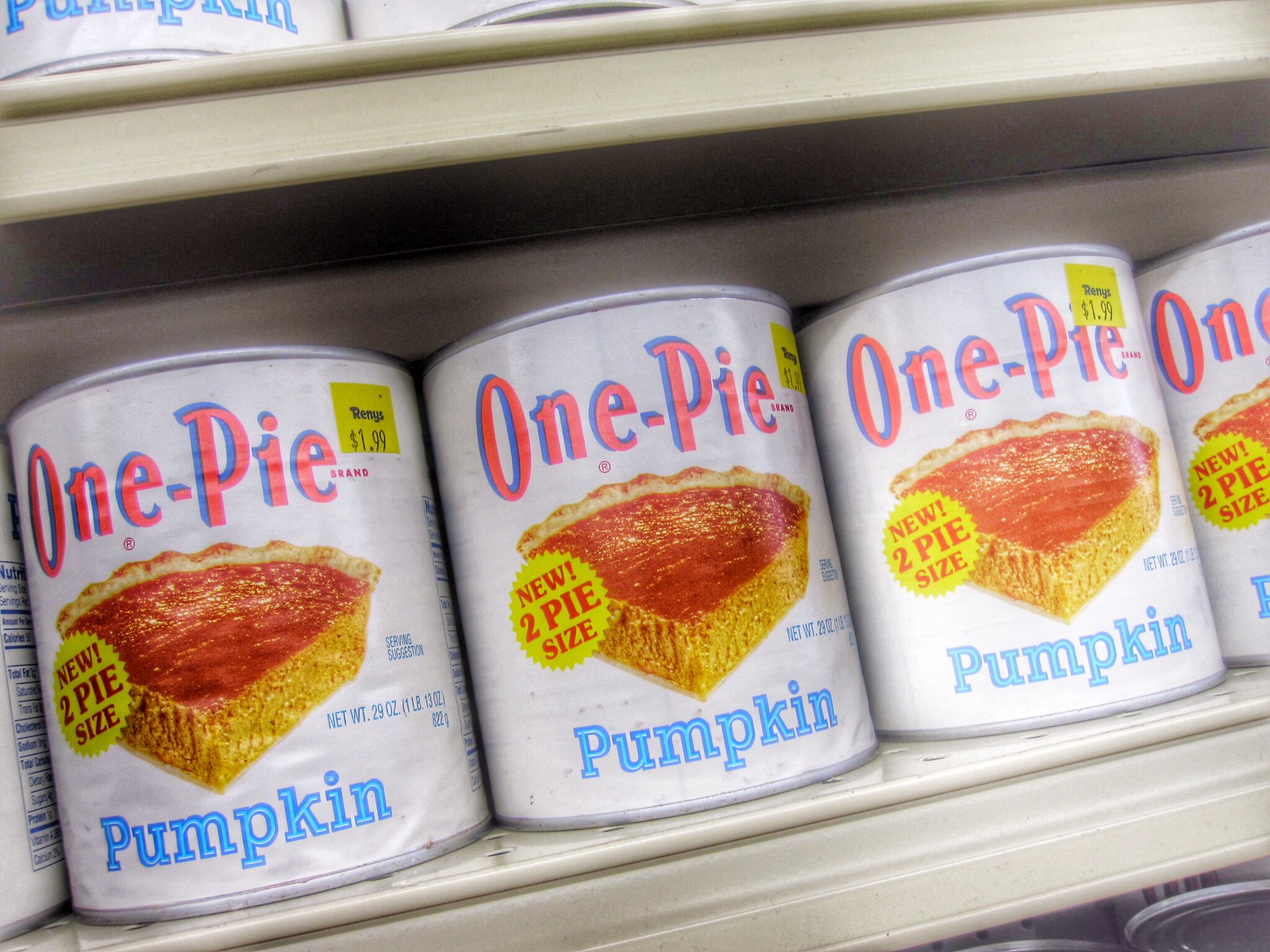This color photograph depicts an old-style supermarket shelf filled with white tin cans of pumpkin pie, likely from the 60s or 70s. The shelf, with creamy greyish edges, holds a row of five cans, three fully visible and two partially shown at the corners. Each can prominently displays an image of a slice of pumpkin pie with red and yellow hues. The label on the can reads "One Pie" in large red text outlined in blue, and "Pumpkin" beneath it in blue. A yellow circle to the left of the pie image announces "New Two Pie Size" in red. The price sticker, in yellow with black text, lists $1.99. The lids are the type requiring a can opener. The net weight of each can is 29 ounces. The entire scene captures the nostalgic essence of a bygone retail era with its basic yet colorful design.